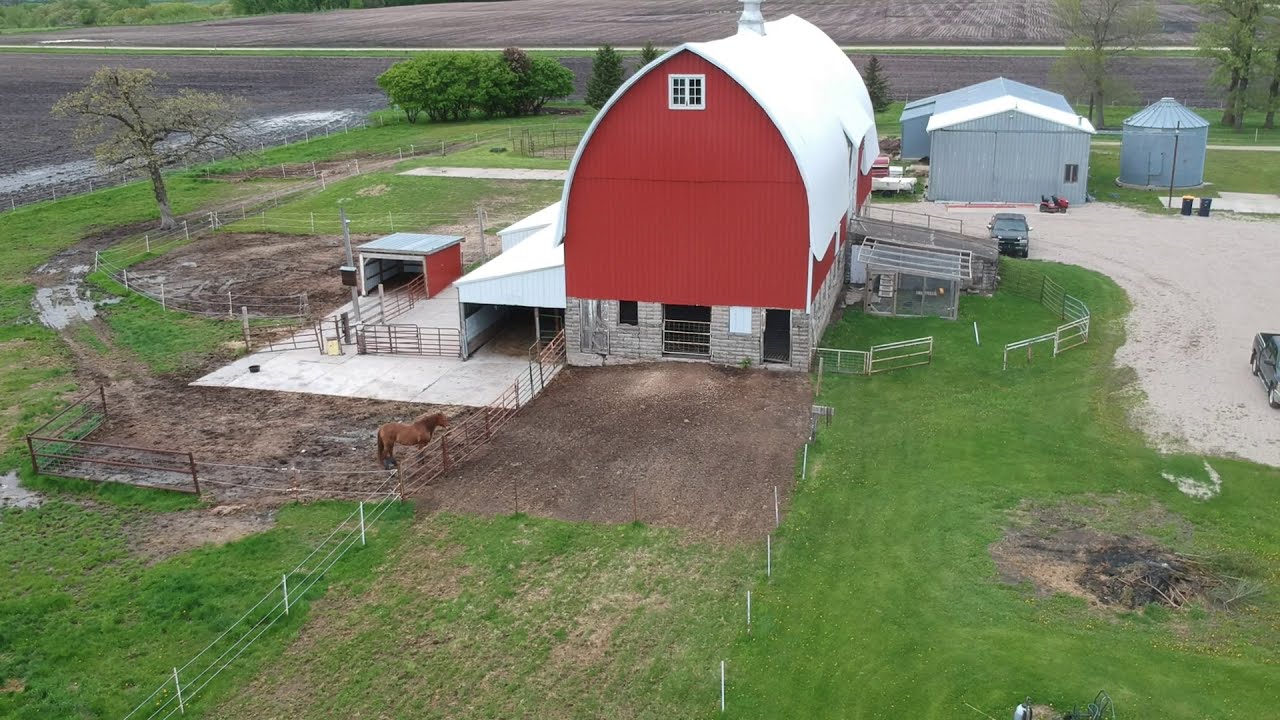This aerial shot captures a vibrant farm landscape centered around a prominent red and white barn, characterized by its unique curved roof and stone foundation. The barn, painted red with a white roof and a distinctive window at its peak, is surrounded by a network of fences and pens. On the left side, a horse stands in a muddy enclosed area, bordered by layers of fencing and a concrete section with large gates. Surrounding the barn are patches of green grass and brown, muddy terrain, with a tree to the far left and a freshly tilled, dark-colored field extending towards the background.

To the right of the barn, a gravel driveway leads to a grayish-blue building and a smaller metal structure, likely used for grain storage. This area also features a burn pile, a few dark-colored trucks, and some farm equipment, including what appears to be a piece of a lawnmower or red farm machinery. Scattered trees and bushes provide a subtle backdrop of greenery against the predominantly earthy tones of the farm.